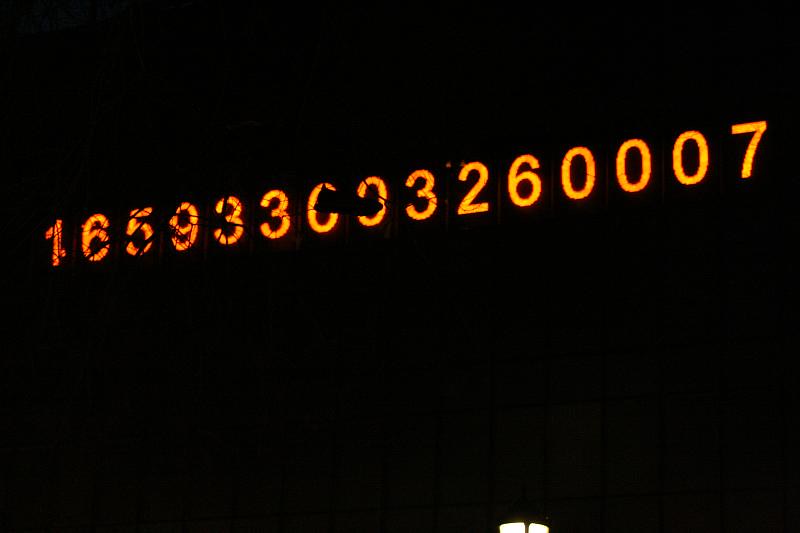The image features a long series of numbers, "165933003260007," displayed in a bright orange font against a stark black background. The screen displaying these numbers appears to be damaged, as evidenced by several black fracture marks disrupting the numerical sequence, suggesting a cracked surface. Alternatively, these dark lines could be interpreted as tree branches silhouetted against the numbers, but the pattern more accurately resembles a broken screen. At the bottom of the image, slightly offset to the right of the center, there are two small, white lights whose purpose or origin is unclear. The overall effect is a striking contrast between the vibrant orange numbers and the deep black and fractured elements of the background.